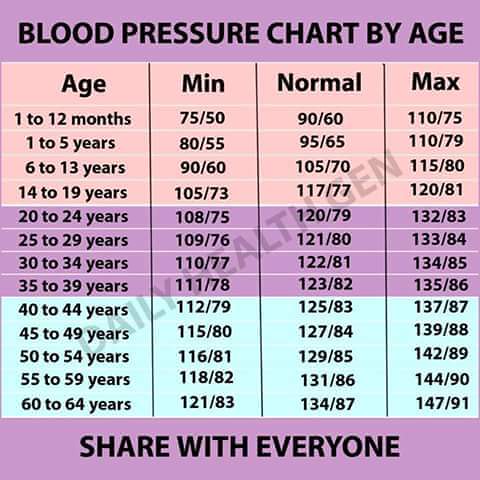This image features a detailed blood pressure chart by age, with a distinct purple border at the top and bottom. The top border prominently displays the title "Blood Pressure Chart by Age" in large black letters, while the bottom border states "Share with Everyone." The chart itself is divided into four vertical columns labeled "Age," "Min," "Normal," and "Max." 

The age groups are divided into color-coded sections: the first four age groups (1-12 months) are set against a peach background, followed by the next four age groups (ages 20-39) on a light purple background, and the last five age groups (ages 40-64) on a turquoise background. Each age group lists corresponding minimum, normal, and maximum blood pressure values. For instance, for ages 1-12 months, the minimum blood pressure is 75/50, normal is 90/60, and the maximum is 110/75. For ages 40-44, the minimum is 112/79, normal is 125/83, and the maximum is 137/87. Vertical black lines separate each column, enhancing the chart's readability. This structured and colorful presentation aims to provide clear and accessible information on blood pressure ranges for different age groups.